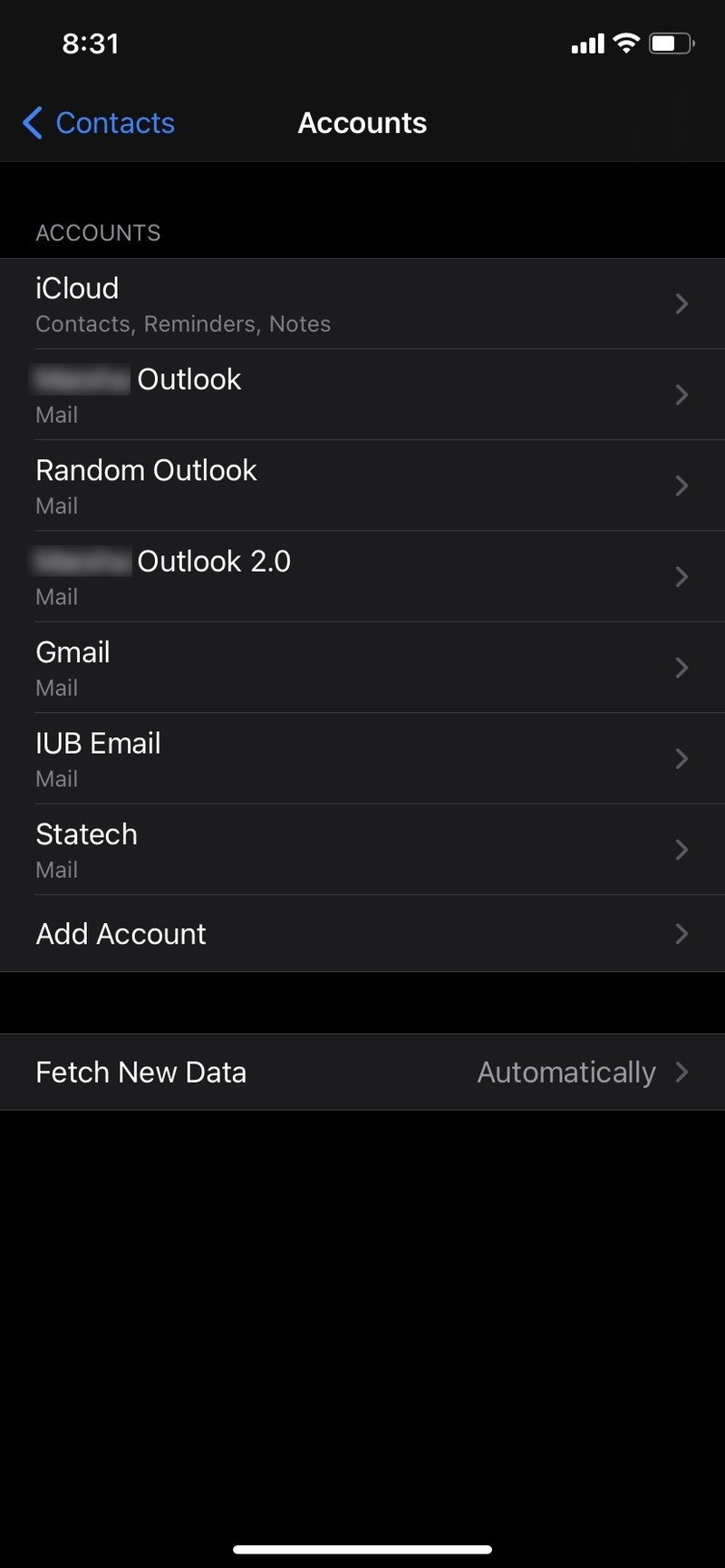This is an image of an iPhone screen displaying the "Accounts" section in the iCloud settings. At the top of the screen, it is 8:31, although it doesn't specify AM or PM. The screen also shows two signal bars, Wi-Fi connectivity, and the battery level in a charging state. 

The page specifically highlights "Contacts" in blue, and "Accounts" in white, indicating that the user is likely within the "Accounts" settings. Below this, various account options are listed, including:

1. "iCloud" - which encompasses Contacts, Reminders, and Notes.
2. Several "Mail" options including a blurred-out item likely related to a generic email account, a "Random" mail account, another blurred-out item, "2.0 Mail," "Gmail," "Random Mail," "IUB Mail," "Test Mail," "Tech Mail," and an option to "Add Account."
3. "Fetch New Data" is shown at the bottom of the list, indicating that the data fetching settings are applied across these accounts.

This image showcases the typical layout and options available within the iCloud settings on an iPhone, focusing on managing contacts, reminders, notes, and various mail accounts configured on the device.